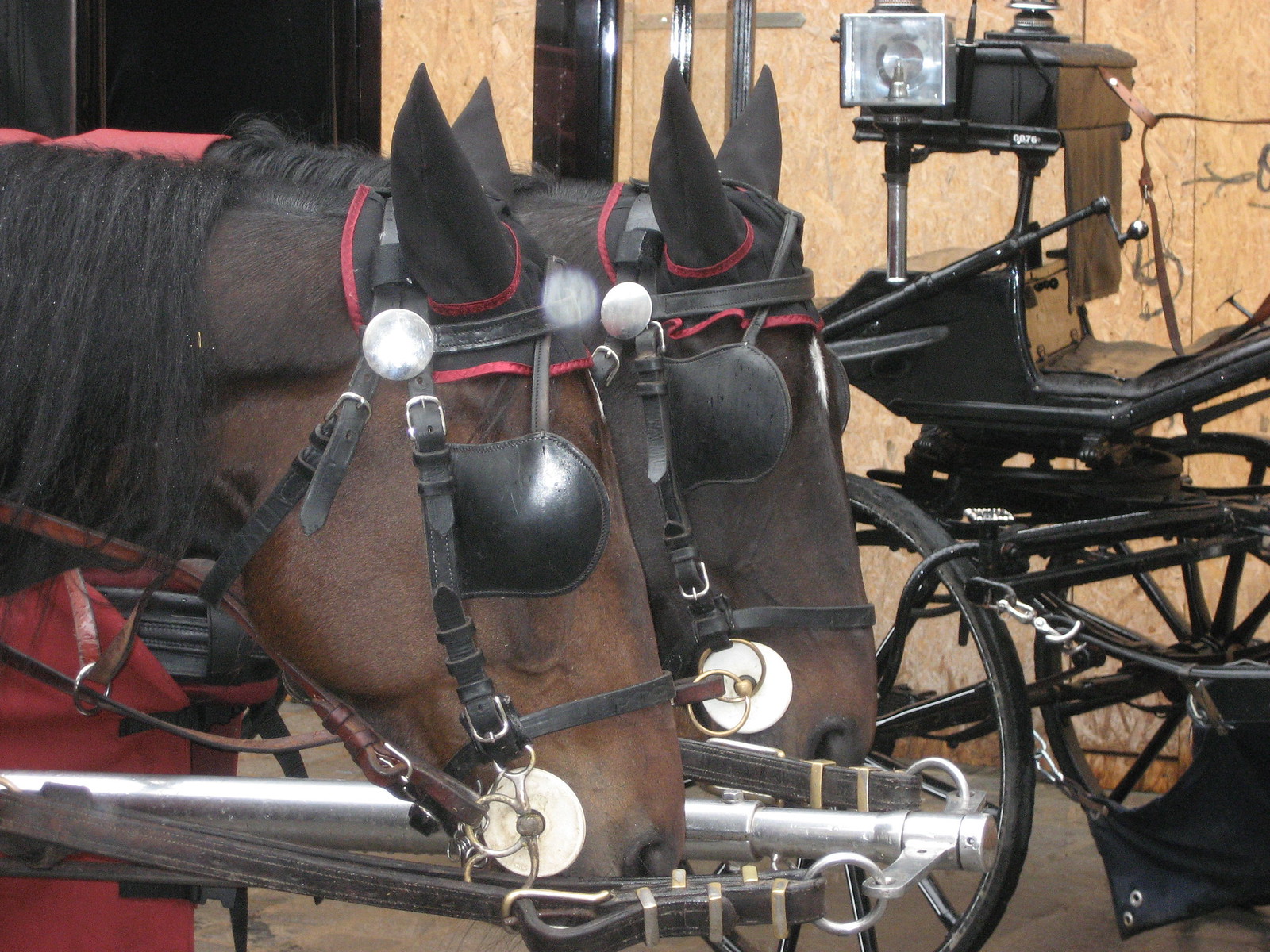This is a detailed close-up photograph of two brown horses with black manes, both fitted with black blinders that limit their view range to just straight ahead. The horses are only visible from the head and neck, stretching in from the left side of the image, facing right, and their ears pointed straight up, covered in black material. They are adorned with black harnesses, detailed with silver buckles, and a red rope or string around their foreheads and ears. The horses appear to be attached to a carriage, although we cannot see the carriage they are pulling. In the background to the right, there's a black metal buggy with black wheels and a small black seat, set against a brown wall and standing on a concrete floor. The photo is taken in daylight, highlighting the dark brown color of the horses' coats and the red blanket visible on them, partially cut off at the bottom left of the image.